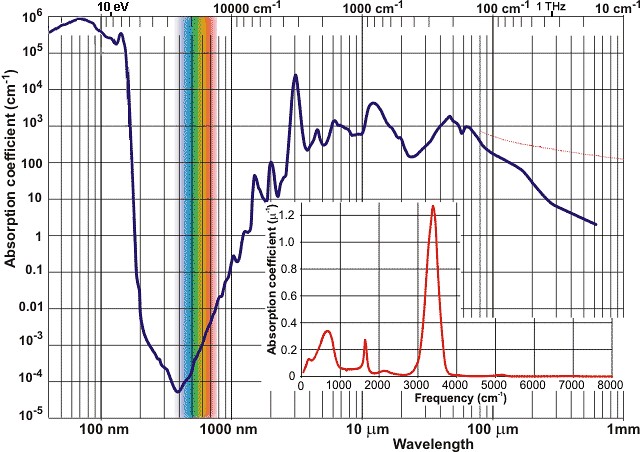This is a detailed and complex rectangular computer-generated graph depicting the relationship between wavelength and absorption coefficient. The x-axis is labeled "wavelength," ranging from 100 nanometers (nm) to 1 millimeter (mm), and the y-axis is labeled "absorption coefficient" in centimeters to the minus 1 (cm⁻¹), spanning from 10⁻⁵ to 10⁶. The graph features numerous vertical lines, including a prominent band of rainbow-colored lines indicating specific wavelengths. Additionally, there are two fluctuating horizontal lines: the top one in dark blue and the bottom one in red. The red line is part of a smaller, secondary graph embedded within the main graph. This nested graph adds another layer of complexity, reinforcing the detailed data captured in this visualization. Overall, the chart is intricate, demanding specific knowledge of nanometers, wavelengths, and absorption coefficients to fully interpret its nuances.